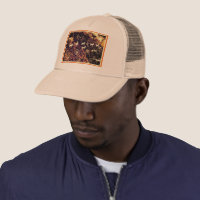This photograph features an African American man wearing a beige or cream-colored baseball cap. The cap has a yellowish-gold, almost square medallion on the front, adorned with a multi-colored design incorporating darker shades like black, orange, and brown. The sides of the cap appear to have a gray panel or mesh for ventilation. The man sports a short beard and mustache. His face is angled downward to the bottom left of the image, making his eyes indistinguishable under the cap’s brim. He is clad in a zipped-up jacket, described variably as navy blue or purple, with a patterned white shirt peeking out from underneath. His pose is square with the camera while his head is slightly tilted, creating an intriguing composition.